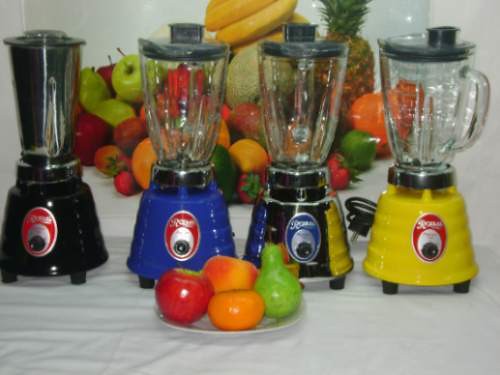This vividly colorful photograph captures a vibrant kitchen scene featuring four blenders positioned in a row on a white tablecloth. Each blender is the same size but distinguished by its colored base: black, blue, silver, and red. The blender bases feature an oval in the middle—three of them with red and silver, while the silver one has a blue accent.

In front of the blenders, a white plate showcases a collection of lifelike plastic fruits: an apple, a peach, a small orange, and a green pear. Behind the blenders, a large tray is brimming with an array of fresh fruits, including bananas, a cantaloupe, a pineapple, green and red apples, oranges, limes, strawberries, and tangerines. The arrangement and assortment of fruits, combined with the colorful blenders, creates a bright and cheerful atmosphere.